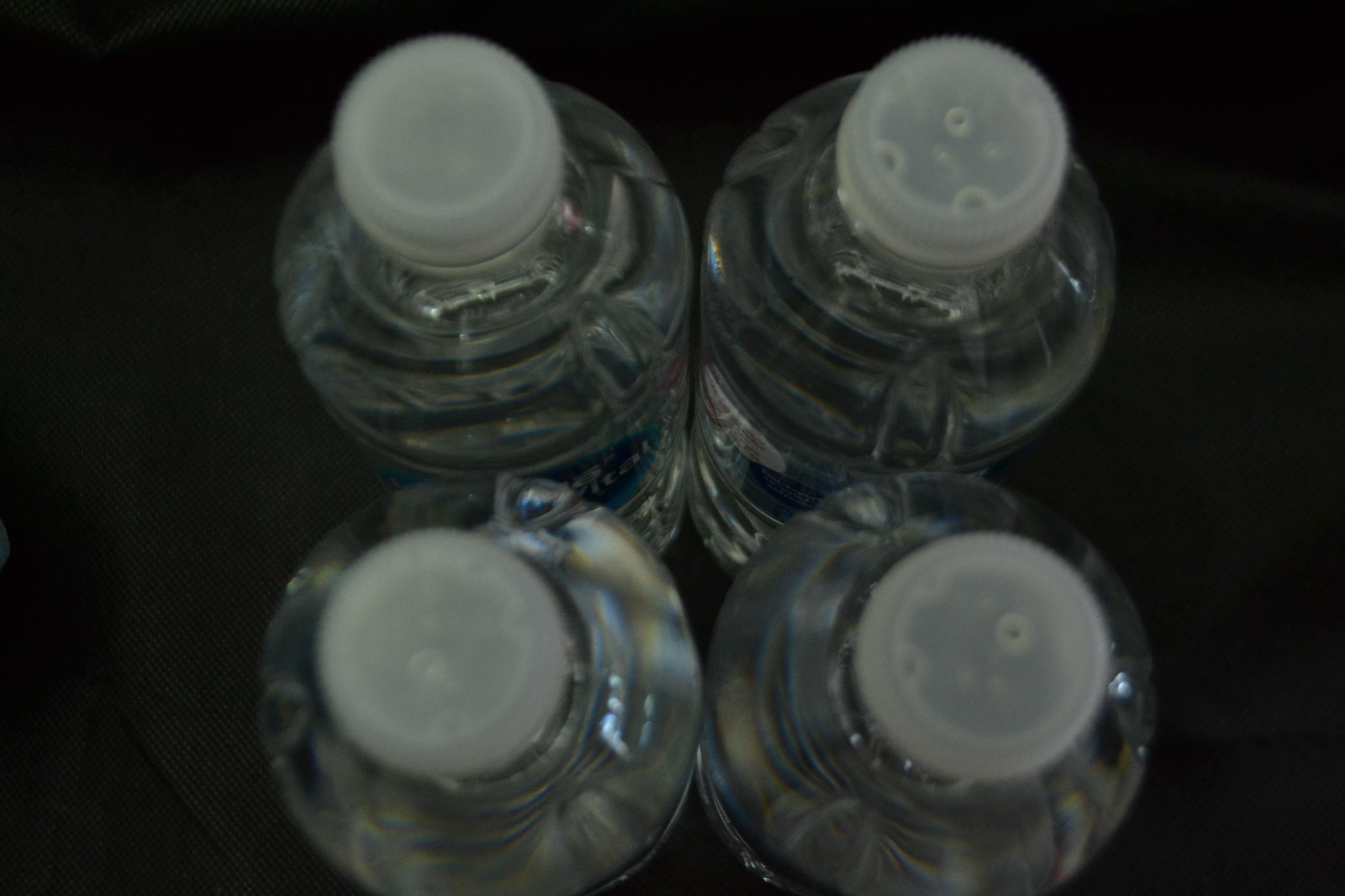The image presents an overhead view of four transparent plastic water bottles, tightly clustered together in a square formation against a textured black cloth background. The bottles are filled to the brim with water, evidenced by the presence of small bubbles within the clear, semi-transparent screw caps. The labels on the bottles are somewhat visible, one displaying a familiar design with a light blue label and white writing, potentially showing the partial text "I-C-A-L." Despite the lack of clear visibility of the labels' details, hints of white and burgundy text are discernible. The bottles exhibit intentional indentations around the top part, likely a characteristic of their manufacturing design. The light refracting through the water and plastic creates irregular reflections, enhancing the simplicity and focus of the image.